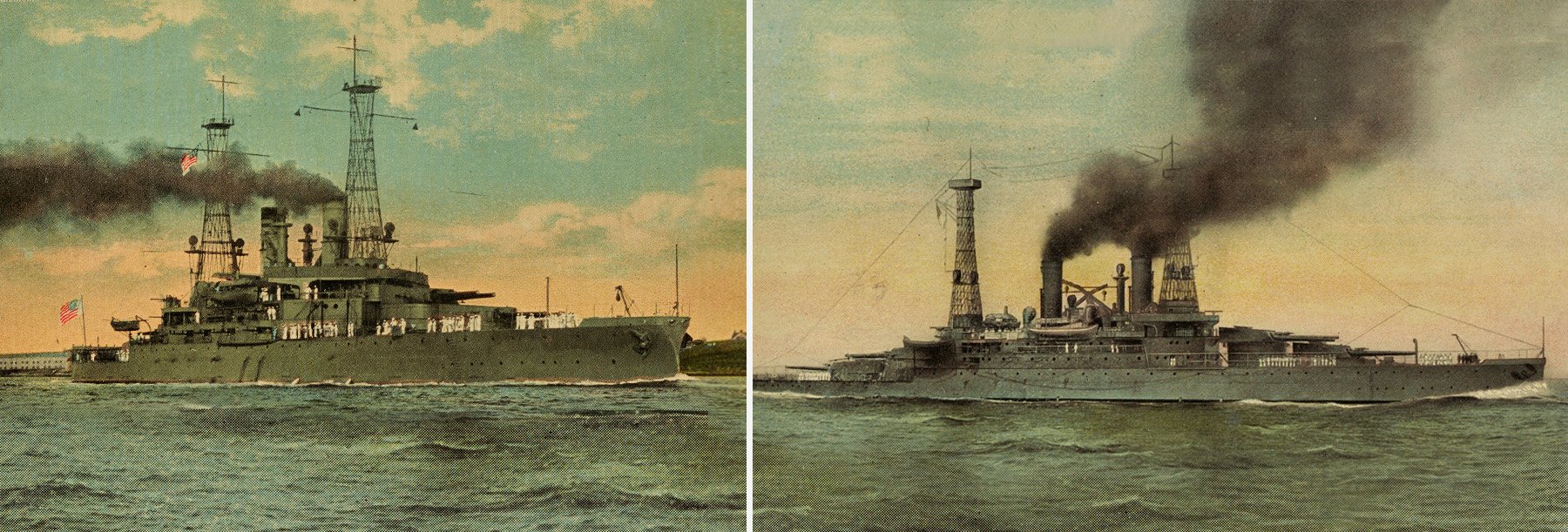The side-by-side images feature two distinct World War II-era battleships, each captured in horizontal rectangles. The vessels are painted in army green and gray tones, adorned with various machinery, antennas, and what appear to be radar screens. Billowing black smoke engulfs the scene, contrasting with the cloudy, somewhat overcast sky, which shows patches of blue and hints of a pale, faded gray. The left ship prominently displays an American flag, while the right ship lacks any flags and has a noticeably longer, pointier front. Both ships, outwardly old and covered in smoke, are unique in their construction and surroundings. The leftmost ship appears slightly closer to land, while the right is more out to sea. Despite some visual similarity, the differences in ship design and the varying sky colors—a brighter sky tinged with yellow and orange on the right, and a more somber, cloud-filled sky on the left—highlight the distinctive nature of each ship. The images suggest they might be retouched photographs or detailed paintings, as the small human figures, if any, are merely specks amidst the vast metallic structures.